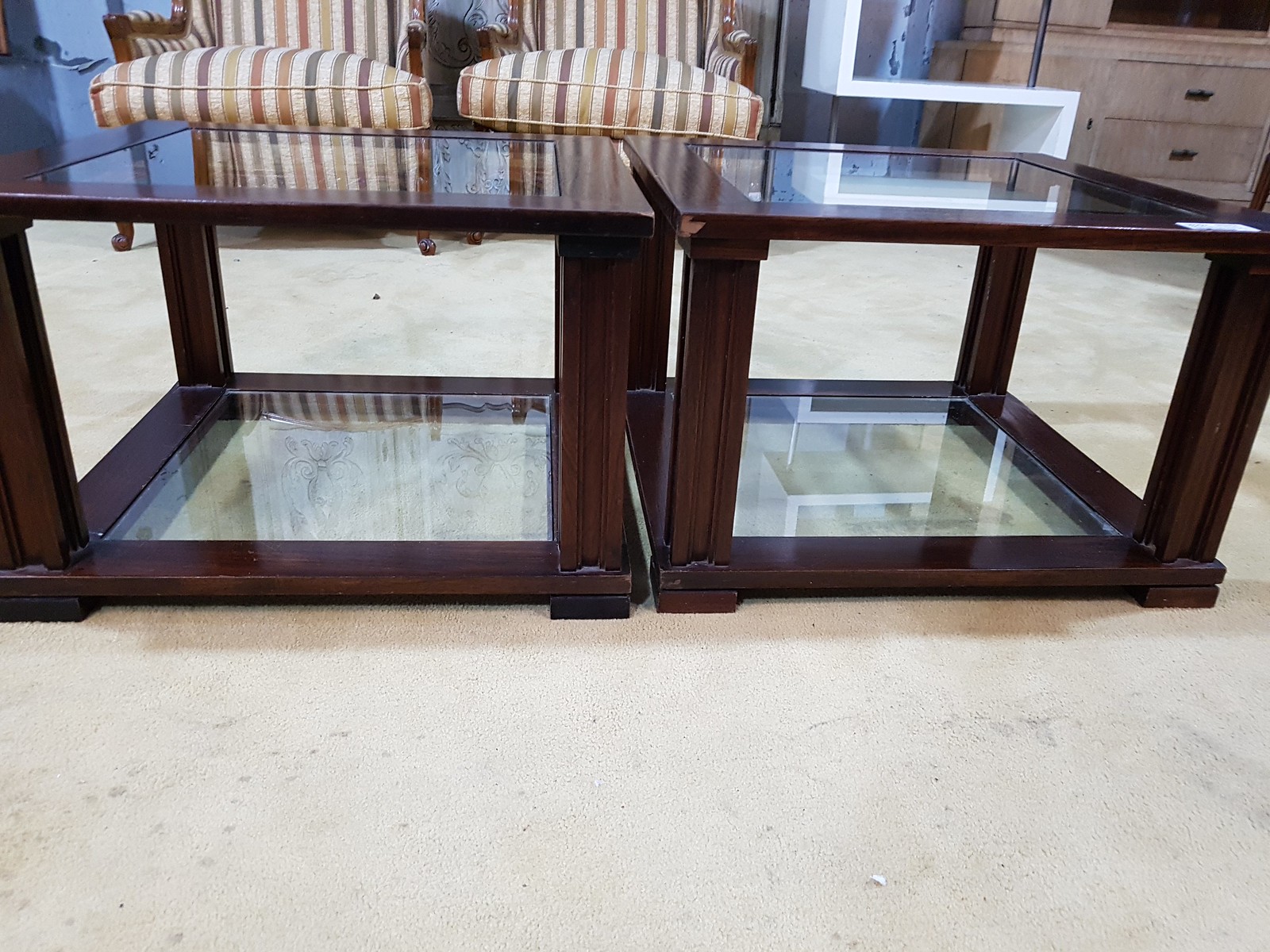The photograph captures a cozy living room setting with a soft, pale-colored carpeted floor. Dominating the foreground are two square, dark mahogany coffee tables featuring glass tops and bottoms, which create a see-through effect. Toward the back of the room, two armchairs adorned with vibrant, vertically striped cushions in colors ranging from red to purple sit neatly side by side. Adjacent to the armchairs, on the right upper corner, stands a light-colored pine wood cabinet, possibly serving as a TV stand, although the top edge is cropped out of the frame. The scene blends warm wood textures with colorful fabric patterns, creating an inviting and eclectic atmosphere.